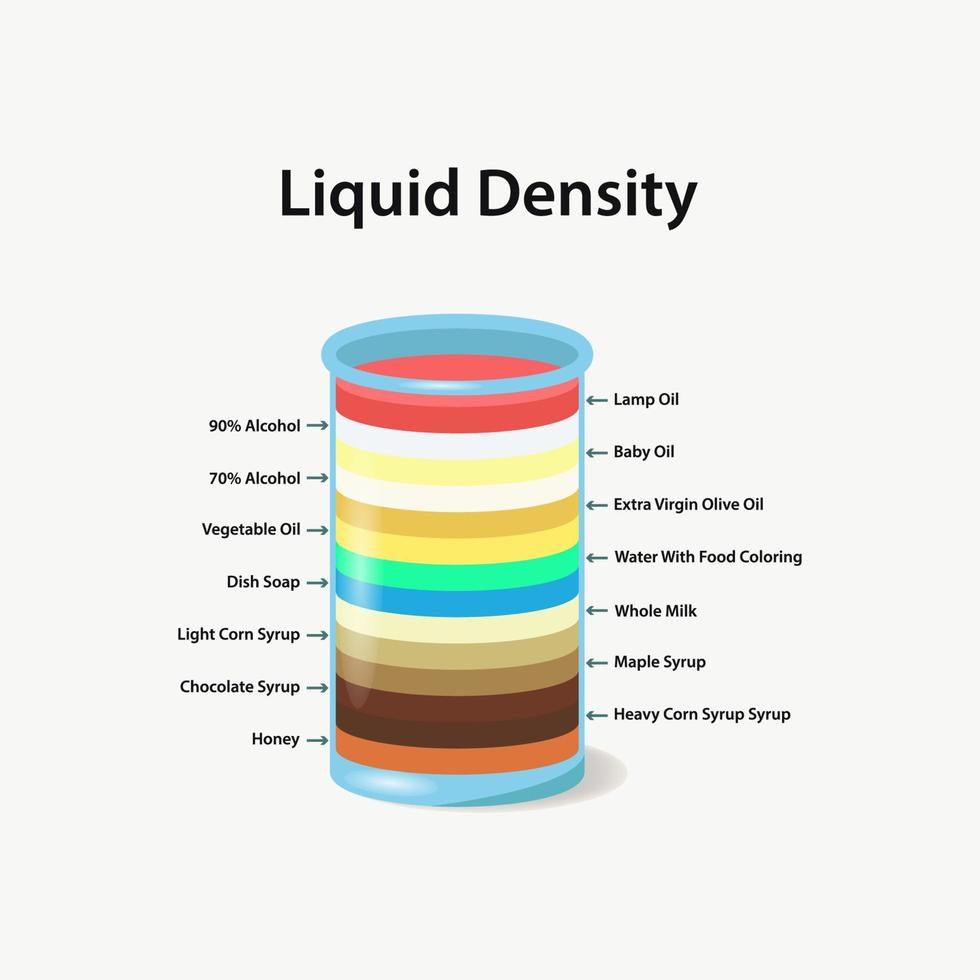The image is a detailed scientific illustration titled "Liquid Density," set against a very light grey background. It features a purely animated, transparent blue cylinder, like a beaker or measuring cup, filled with various colored liquid layers, each representing different densities. The liquids are labeled with black text and arrows pointing to their respective layers. 

From the top:
1. **Lamp Oil** — A red layer.
2. **90% Alcohol** — A white layer.
3. **Baby Oil** — A pale yellow layer.
4. **70% Alcohol** — Another white layer.
5. **Extra Virgin Olive Oil** — A tannish brown layer.
6. **Vegetable Oil** — A lighter yellow layer.
7. **Water with Food Coloring** — A vibrant green layer.
8. **Dish Soap** — A blue layer.
9. **Whole Milk** — A pale yellow layer.
10. **Light Corn Syrup** — A beige layer.
11. **Maple Syrup** — A dusty brown layer, slightly darker than the previous.
12. **Chocolate Syrup** — A rich chocolatey brown layer.
13. **Heavy Corn Syrup** — A darker brown layer.
14. **Honey** — A muted orange color at the very bottom.

The layers appear to be in equal volumes, displaying their varying densities. The cylinder is illustrated in a bluish hue, and the overall minimalist design presumably targets educational purposes, potentially for a textbook.